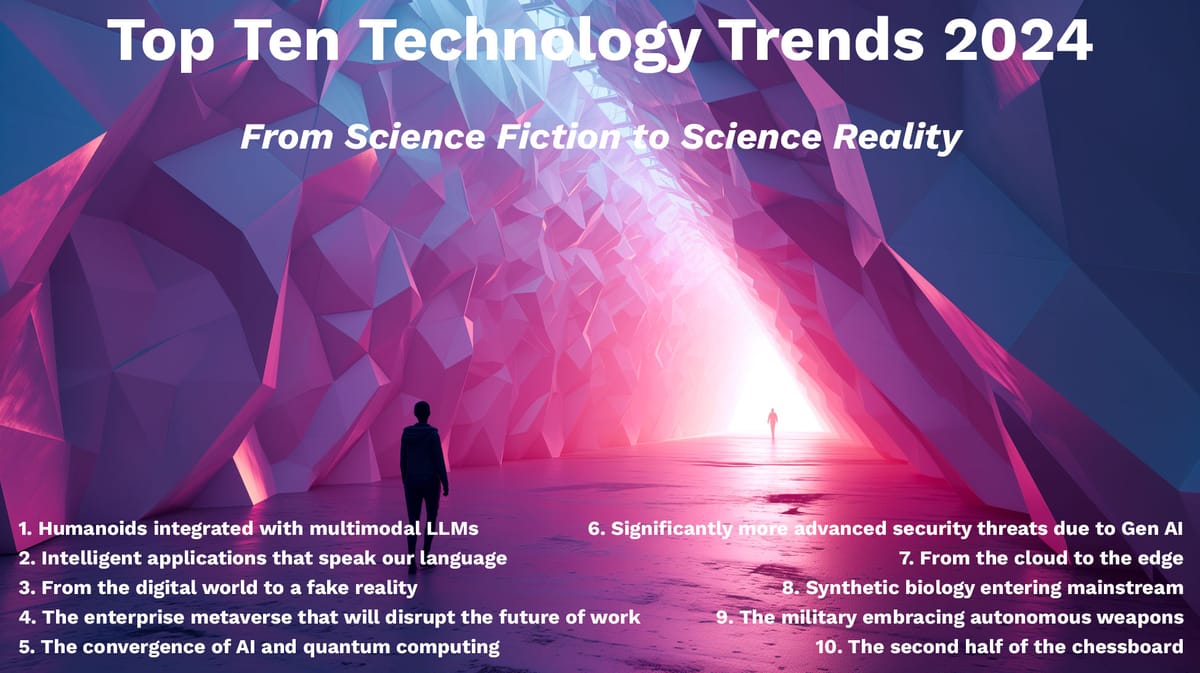This colorful illustration, reminiscent of a presentation slide or YouTube thumbnail, showcases the "Top Ten Technology Trends 2024: From Science Fiction to Science Reality." The scene features a cave-like opening with a complex geometric ceiling of hexagons and triangles, transitioning from bluish tints in the foreground to hues of pink and purple with white light in the distance. Two silhouetted figures, one near the bottom left and another barely visible at the far end, add a sense of human presence. The cave's interior and exterior crystals further enhance its futuristic ambiance. Text at the top lists the main title and subtitle, while the bottom features two columns numbered one through ten, detailing trends like humanoids integrated with multimodal LLMs, AI and quantum computing convergence, and the rise of synthetic biology and autonomous weapons. The overall effect combines vivid colors and advanced technological themes to illustrate the future of innovation.